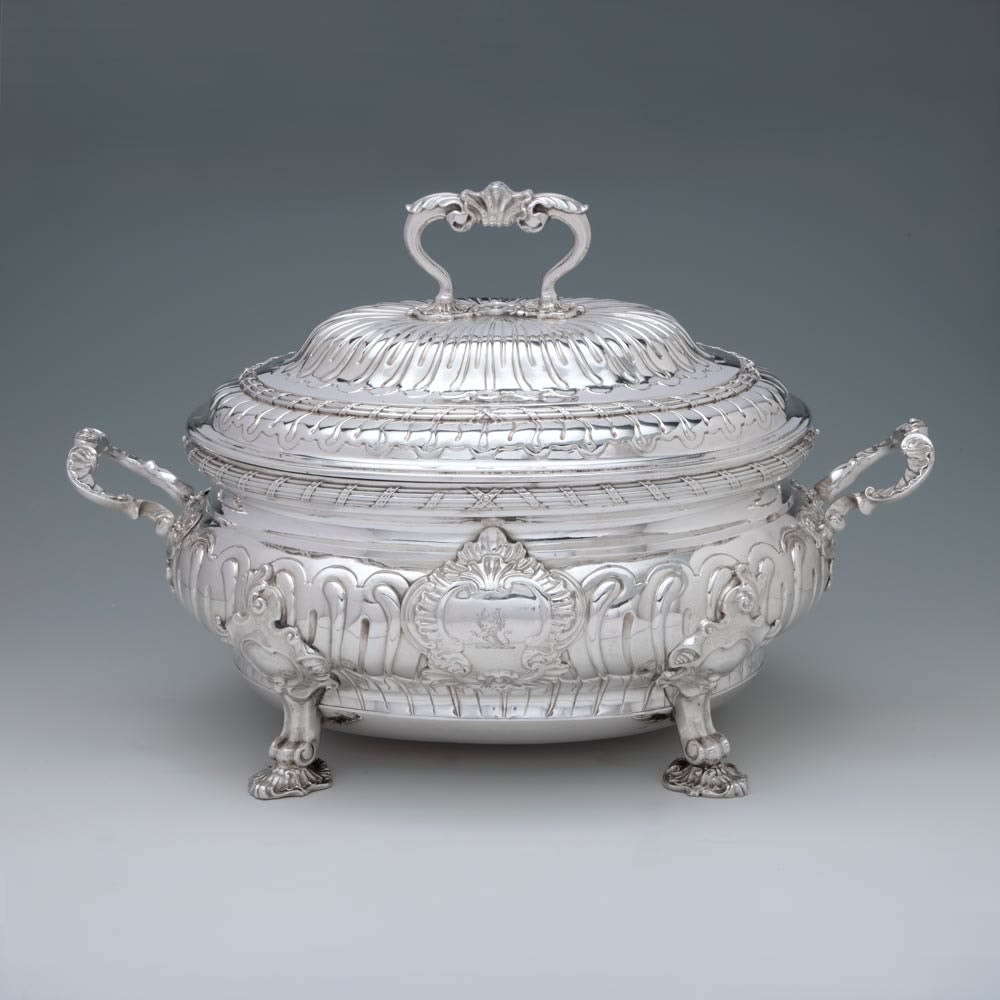The image features a square photo with a background that transitions from darker gray at the top to lighter gray at the bottom. At the center of the image is an ornate, silver serving tray or cloche, which is made from stainless or sterling silver. The serving tray is highly detailed with an intricate, regal design and possesses a lid topped with a handle. The tray itself stands on four decorative feet, reminiscent of those found on antique clawfoot bathtubs. Additionally, there are two handles on either side of the tray, likely for carrying. The entire composition of the image exudes a silvery, almost white sheen without any brassiness, set against a simple gray background that highlights the luxurious item. The item is oblong and round in shape, with no other identifying marks or objects in the frame.